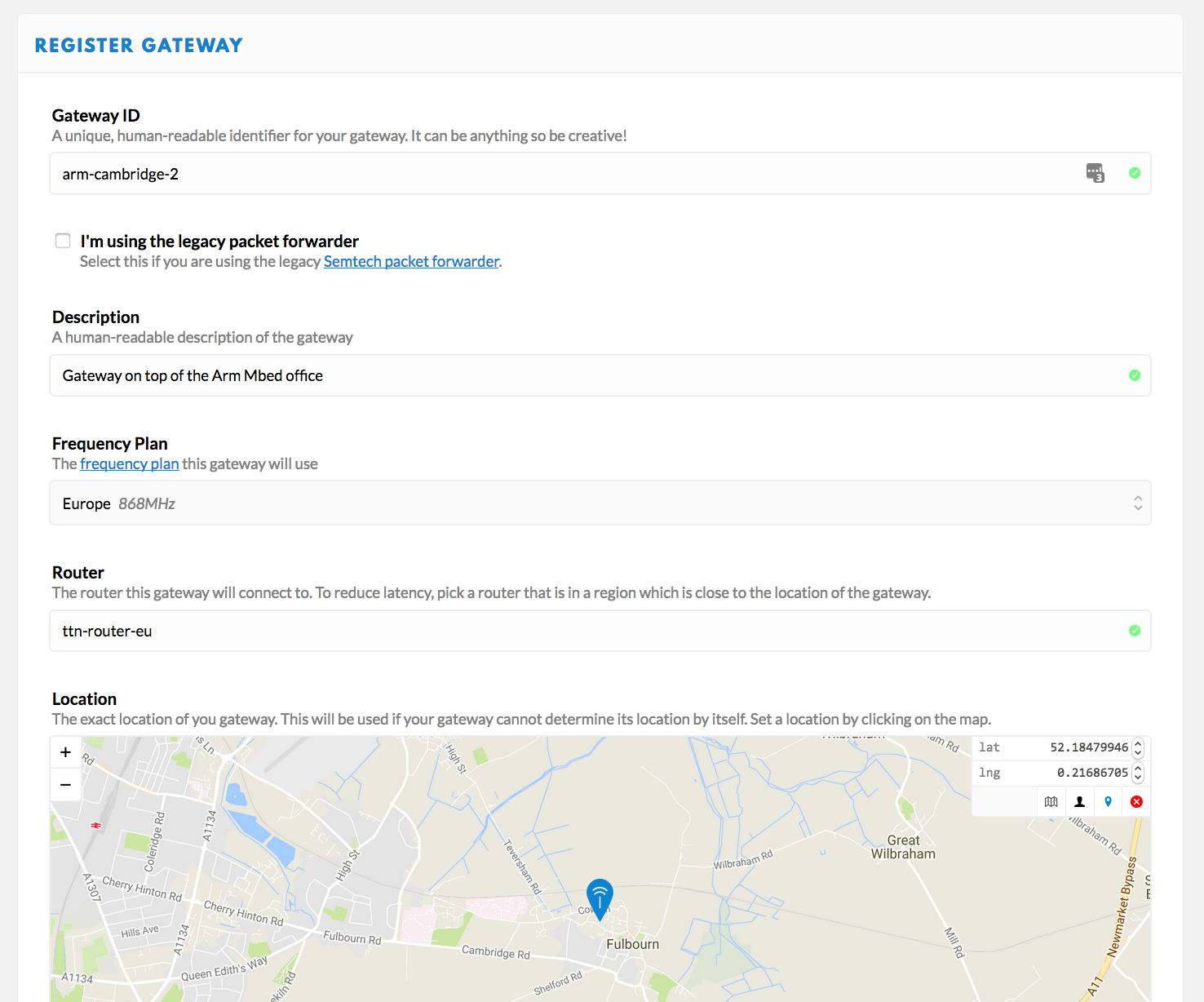This is a detailed caption of the "Register Gateway" webpage from a website. 

At the top-left corner of the page, the website name, "Register Gateway," is prominently displayed. Below this header, the page is divided into various white sections featuring black text, blue hyperlinks, and interactive fields.

The first section includes fields for entering a unique identifier for your gateway, labeled "Gateway ID." The text encourages creativity with the identifier: "You can be anything, so be creative!" Adjacent to the entry box, which contains the example "ARM-Cambridge-2," there is a green circle with a white checkmark indicating validation.

Below the Gateway ID section, there is a checkbox option labeled "I'm using the legacy packet forwarder," which should be selected if relevant. An adjacent blue hyperlink directs users to the "Symtec packet forwarder."

Next is a section for providing a human-readable description of the gateway. The entry box contains the example text "Gateway on top of the ARM mbed office," with another green circle and white checkmark indicating approval.

Following the description, there is a section labeled "Frequency Plan." Users can choose a frequency plan for their gateway from a dropdown menu, with the selected option being "Europe, 868 MHz." A blue hyperlink likely provides more information on frequency plans.

Further down is the "Router" section, where users can select a router for their gateway to connect with. It advises selecting a router located in the same region as the gateway to reduce latency. The entry field shows "TT-router-EU," with a green circle and white checkmark indicating it has been correctly selected.

At the bottom of the page, there is a map showing the exact location of the gateway. Users can set this location manually if the gateway cannot determine it automatically. The map provides an interactive feature where the user has clicked to set the gateway's location.